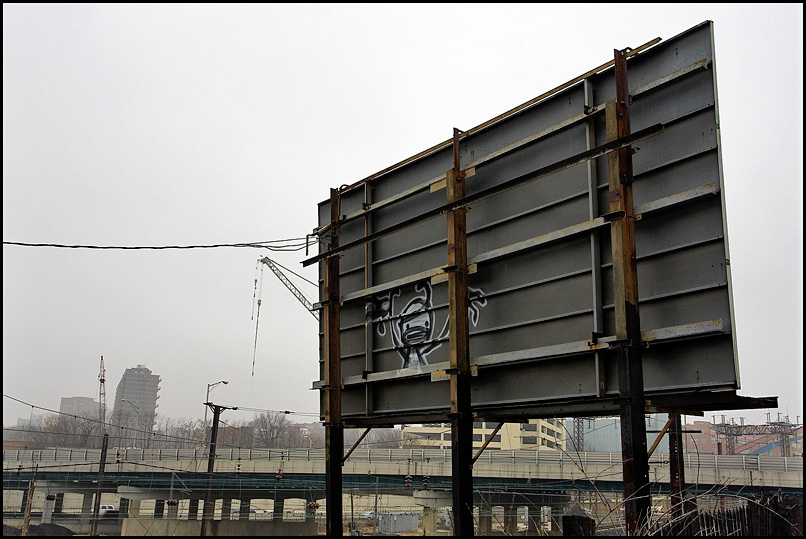The color photograph captures an outdoor urban scene under a gray, overcast sky, indicating it's likely wintertime. Dominating the foreground slightly right of center is the back of a billboard, supported by rusting beams. The metallic backside of the billboard features a graffiti of a stick figure with arms raised, rendered in white and black to creatively mimic prison bars using the ridged surface. An elevated highway cuts through the middle of the image, its green girders and beams supporting a concrete top with white railings. In the background, two lifeless, leafless trees flank two buildings on the left, while construction cranes and numerous telephone wires span across the hazy backdrop. The scene also includes a tall building and distant structures further emphasizing the urban environment, with the entire composition framed wider than it is tall.